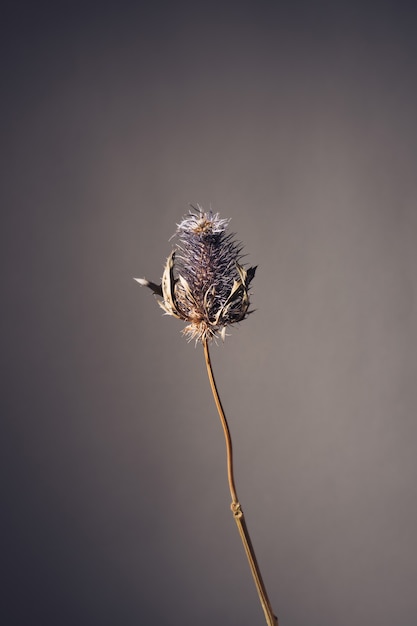This image features a detailed, close-up view of a single dandelion weed against a gradient gray background. The stem of the dandelion, which is long and thin, extends from the very bottom right of center and angles steeply upward to the left, ending just above the center of the image. The background is dark gray around the edges and gradually becomes lighter towards the center, providing a stark contrast that highlights the dandelion. The dandelion appears devoid of its white, fluffy seeds, leaving behind a bare, brown, cone-shaped structure with a slightly feathery appearance towards the top. There's a knuckle-like growth plate midway up the stem. Around this area, some light, dead-looking leaves are visible. Although one description mentions purple spikes and a white feathery look at the base, the predominant shared observations focus on the cone's brown color and remnants of what appears to be a once fluffy dandelion now reduced to its central core structure. The minimalist setting is devoid of any other objects or text, emphasizing the solitary dandelion weed against the somber, gradient backdrop.